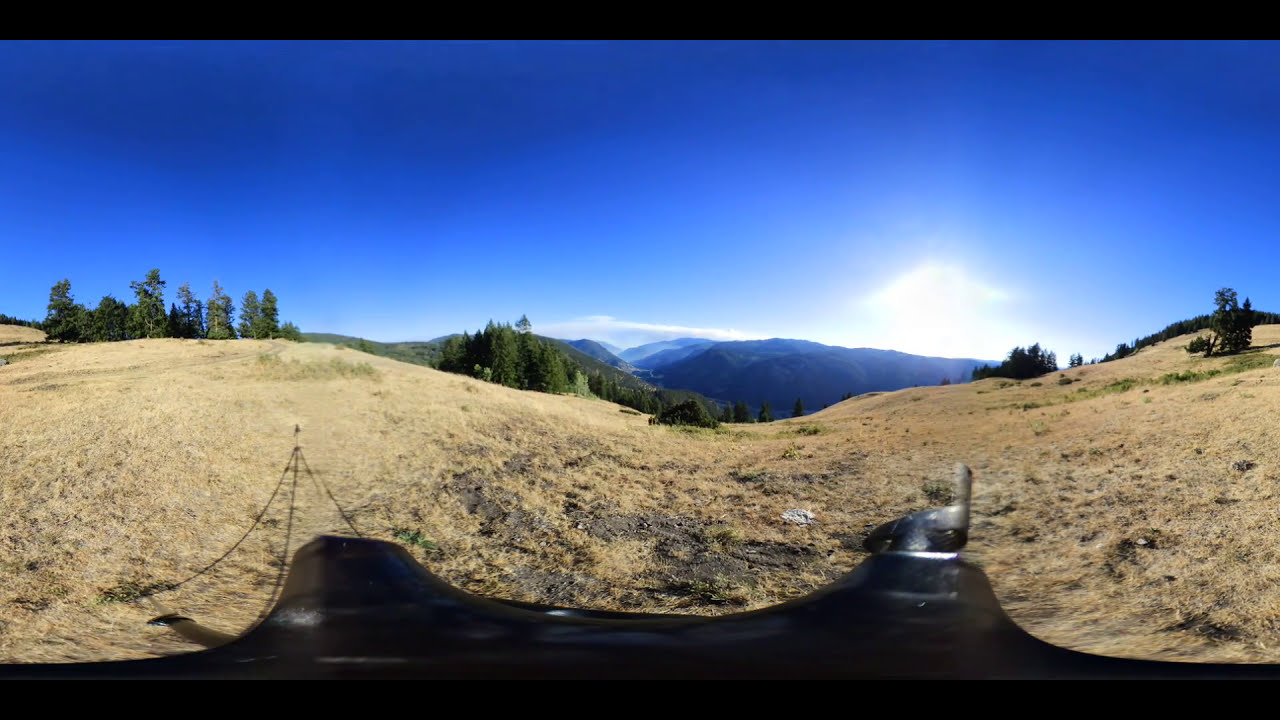In the image, we observe a rugged yet expansive mountain terrain under a bright blue sky with sunlight filtering through occasional clouds. The scene appears stitched together from different photographs, creating a slight curvature in the ground that gives a panoramic view. The landscape starts from a relatively smooth, flat ridge at the top of a hill covered mostly in yellowing, dead grass, interspersed with patches of green. To the left side of the ridge, there is a cluster of trees of varying heights: short trees in the middle, tall trees on the left side, and medium-sized trees at the far left end. 

Further in the distance, more mountain ridges loom, appearing darker and almost black due to the sunlight hitting them, with the farthest ridges showing hints of white, possibly from snow. A vehicle, perhaps silver and black in color, driven by an individual, can be seen navigating the undulating terrain, moving towards the greener patches of trees and the distant mountains. The sky remains clear and blue above the observer’s vantage point but hints at a potential storm over the mountains to the left.